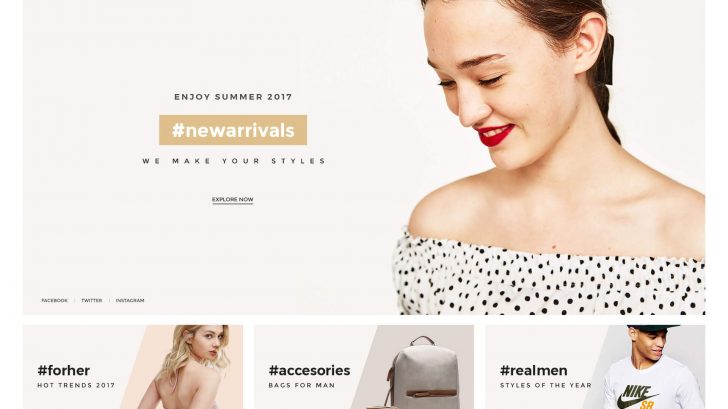The screenshot captures a website dedicated to selling clothing for both men and women. Dominating the visual space is a large banner image set against a very light beige background. On the right side of this banner is a photograph of a woman, captured from mid-chest upwards but with the top of her head slightly cut off. She has light skin, reddish hair tied behind her neck, and is adorned with bright red lipstick. Her attire consists of a white off-the-shoulder shirt dotted with small black polka dots. She is angled slightly away from the viewer, her gaze directed downwards towards the center of the page. 

To the left of her image, the text "Enjoy Summer 2017" is prominently displayed. Beneath this, a darker beige-colored rectangle features the text "#NewArrivals" in white. Below this, in black text, it reads "We make your styles," accompanied by a link labeled "Explore Now."

At the bottom of the screenshot are three smaller banners arranged from left to right. The first banner on the left showcases a young blonde woman seen from behind, barely clad, with the text "#ForHer Hot Trends 2017" adjacent to her. The center banner features the text "#Accessories Bags for Men" and displays a photograph of a backpack. The rightmost banner depicts a man sporting a Nike T-shirt, alongside the text "#RealMen Styles of the Year."